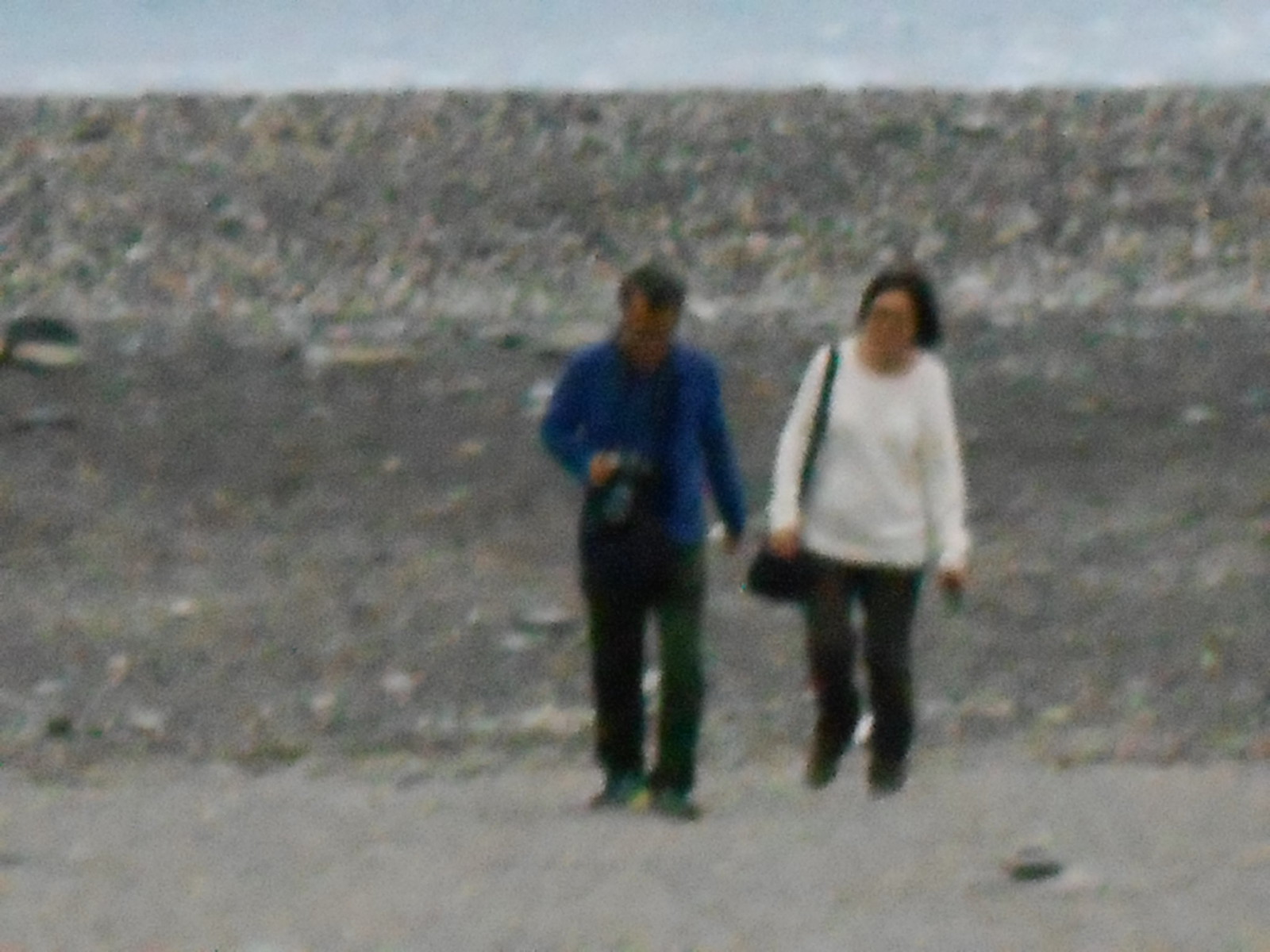In this blurry photograph, two older individuals of Asian descent are walking on a grey, rocky ground that resembles a beach of pebbles or gravel. Positioned in the middle of the image, the man, who is on the left, has a slightly receding hairline with black hair and tan skin. He is dressed in a blue long-sleeved shirt, dark pants—possibly black or dark green—and dark, possibly grey shoes. He is visibly holding a black object, potentially a camera with a large lens, in front of him. Beside him on the right is a woman with a black bob haircut and slightly lighter skin than the man. She is wearing a long, oversized white sweater, black pants, and dark shoes. A black purse hangs from her left shoulder, and she appears to be holding a small object, likely a phone, in her right hand. The background is a gradient of grey tones that lightens towards the top, hinting at a sky but remaining out of focus and hard to distinguish.